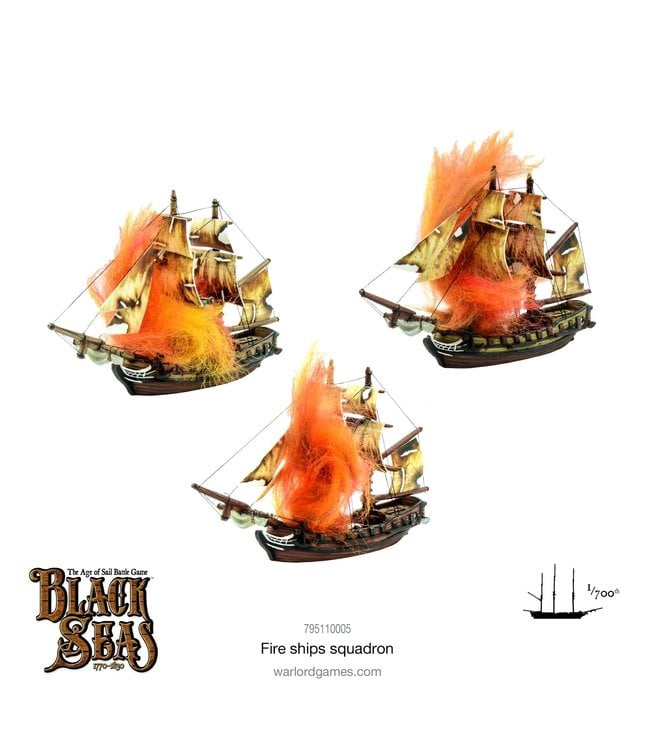This promotional poster for the Age of Sail Battle Game, "Black Seas," showcases three intricately detailed, 1:700 scale model schooners, designed to represent an era spanning from 1770 to 1890. Against a crisp white background, the centerpiece of the poster features three identical, fully-rigged sailing ships with scorched and tattered sails set ablaze by simulated orange and yellow flames, vividly capturing the chaos of naval warfare with "Fire Ship Squadron" emblazoned in black beneath them. Additional text in the lower left corner reads "Black Seas, the Age of Sail Battle Game, 1770-1830," indicating the historical context of the game. The ships, appearing almost like traditional pirate vessels, are meticulously rendered in black with touches of yellow or light tan, adding to their authenticity. At the bottom center, a serial number (795110005) and the website "warlordgames.com" are clearly displayed, while the lower right corner features a basic schematic of a ship and the scale notation "1:700," indicating the miniature size relative to the actual ships. The poster effectively merges historical immersion with gaming excitement.